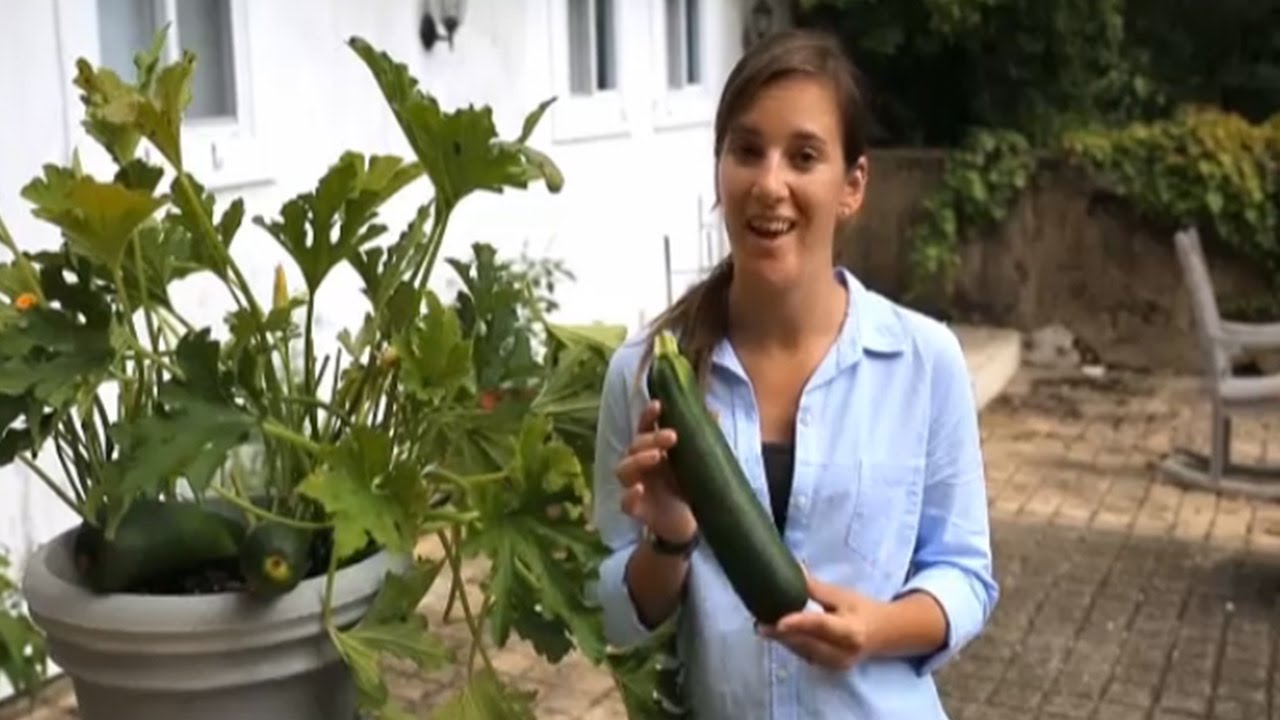In this backyard scene, during daytime, a Caucasian woman, approximately 28-30 years old with dark brown hair tied back in a ponytail, stands on a red stone-paved patio outside a white house. She is positioned centrally in the frame, dressed in a blue button-up denim shirt over a black tank top, and wears a wristwatch. She is holding a large green zucchini with her left hand at the base and her right hand at the top, smiling as though she's describing it to the viewer.

Behind her, the exterior of the house showcases windows on the second floor and a porch area. To her right (our left), a potted plant with wide leaves, likely an elephant ear or similar, is visible, with two more zucchinis growing at its base. The scene is enclosed by a brown wooden fence adorned with dark green ivy. A gray stone planter with additional greenery sits nearby, and a wooden rocking chair is positioned to the right of the frame. The overall atmosphere suggests a slightly overcast day, adding a muted yet warm ambiance to the backyard garden setting.